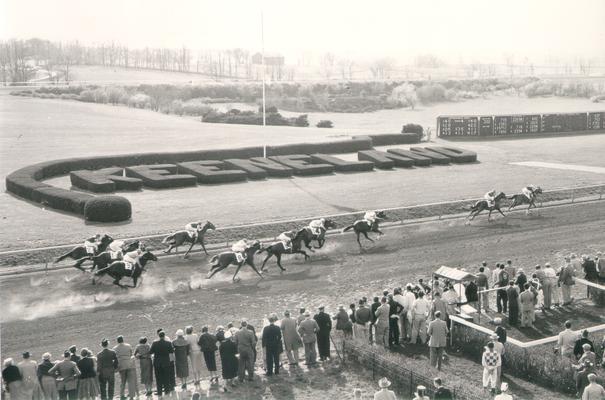This vintage black-and-white photograph captures an exhilarating moment at a horse race, featuring around ten horses mid-race, kicking up dust as they charge forward. Two horses have separated from the pack, leading the race while the others trail behind. A significant number of spectators, dressed predominantly in dark or gray clothing likely from the 1930s to the 1950s, line the front of the racetrack, engrossed in the action. In the bottom right corner, a couple of individuals in jockey uniforms can be seen. Behind the track, the word "Keeneland," crafted from sculpted bushes, stands prominently. The background showcases manicured fields, trees, and rolling hills, adding depth to this historic scene.